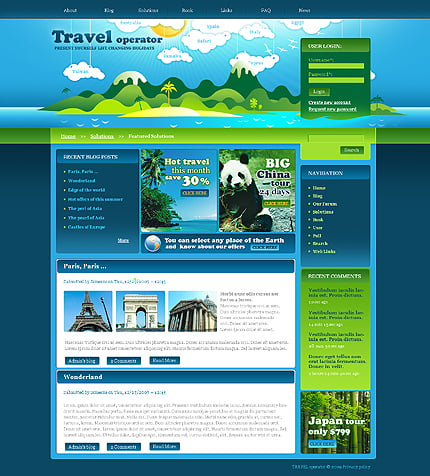This webpage from a Travel Operator features a predominantly sea blue background and is densely packed with information and visuals. The top portion sports the site's name, "Travel Operator," with an image of the sun and floating clouds, accompanied by unreadable text on the clouds. Below this header is a picturesque, cartoonish scene depicting green mountains surrounded by blue waters. As you scroll down, the page is divided into various sections and boxes.

The upper third prominently displays an inviting tropical island image. Moving downward, the layout features three primary boxes: the left box, which is blue with unreadable text; the center box highlights a "Hot Travel Deals" promotion with a 30% discount; and the right box showcases an advertisement for a "Big China Tour" spanning 24 days, illustrated by a panda munching on bamboo. Adjacent to these boxes on the right side is a vertical filtering bar.

Further down, the page reveals more travel destinations, including glimpses of the Eiffel Tower, the Arc de Triomphe, and possibly the Parthenon, although the images are small and somewhat unclear. In the bottom section, additional details become visible, including a "Japan Tour" advertisement priced at $799 with a backdrop of trees. The lower center consists of two large white rectangular sections, the upper one displaying several famous tourist attractions, albeit blurred, and the lower one filled with more unreadable text.